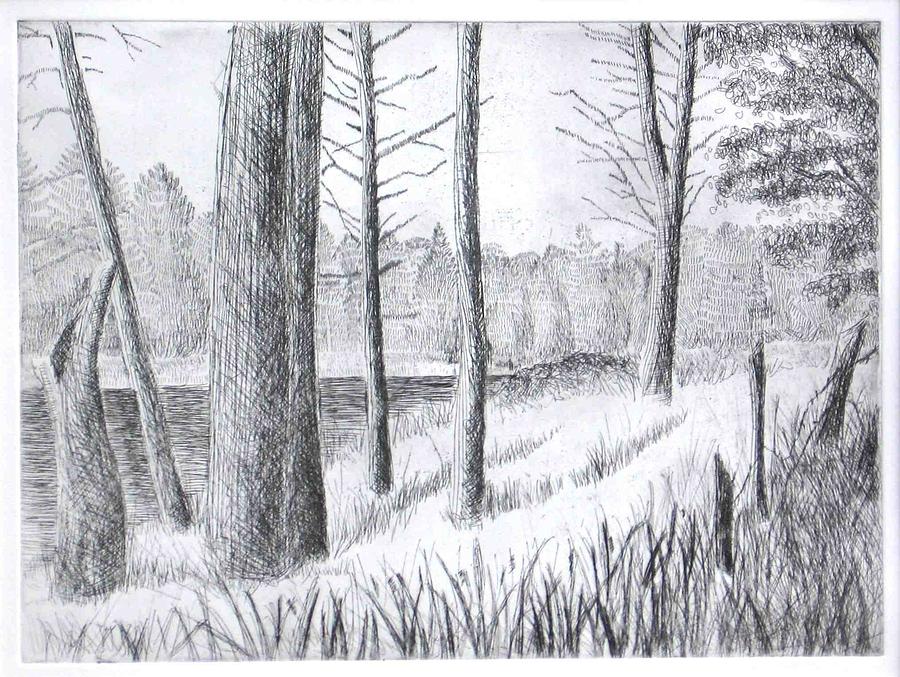This black and white pencil sketch depicts a serene wooded scene featuring a river that winds out of view around a bend. The foreground is dominated by a grassy area with several dead or broken trees, including one that leans with numerous barren limbs. In this area, you can also find at least seven tree trunks, some half-broken, and small sticks protruding from the grass. The artist uses extensive cross-hatching to shade these trees, creating a semi-realistic texture.

The background showcases a forest of evergreen trees whose triangular tops are rendered with tiny lines and pointillism-like techniques to provide depth. The scene displays clear skies which remain pure white, adding contrast to the densely detailed trees and ground. Some leaves can be seen on firs in the background, suggesting they are evergreens. The drawing is possibly framed or bordered by a white outline. The intricate stylistic choices, such as the abundant cross-hatching and delicate line work, highlight the meticulous craftsmanship of this evocative sketch. Additionally, a small fence with metal wire and spikes is faintly visible amongst the grass in the foreground, further enhancing the detailed composition.